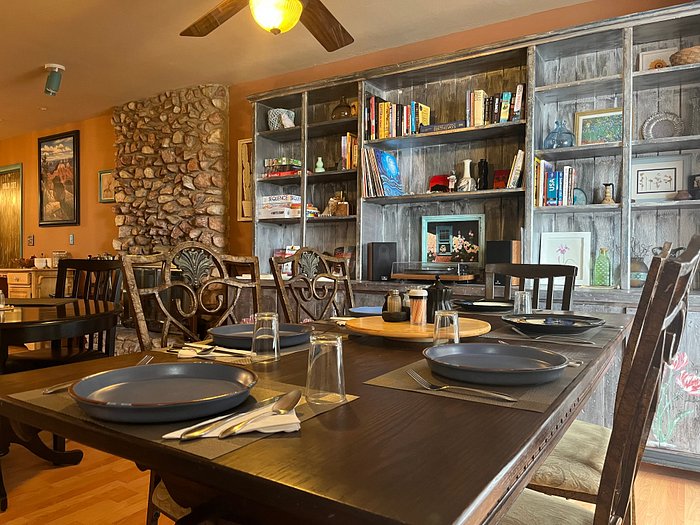The image captures a cozy and detailed dining area inside a home. The room features a wooden floor and is bathed in warm lighting from a ceiling fan with an accompanying light fixture. The main focus is a dark brown rectangular table set for five, each setting adorned with unique gray bowls that have considerable depth. Upside-down glasses, silverware, and neatly folded napkins complete the place settings. At the center of the table sits a wooden Lazy Susan, hosting toothpicks and salt and pepper shakers.

The backdrop reveals a brown wall with an extended gray wood cabinet stretching horizontally, topped with shelves loaded with books, photos, knickknacks, and even a record player with speakers, adding a touch of retro charm. Hanging pictures also accent the wall. Adjacent to the main dining table is a smaller black circular table with black chairs, offering additional seating. The entire space exudes a homely yet meticulously arranged atmosphere, perfect for intimate dinners and gatherings.